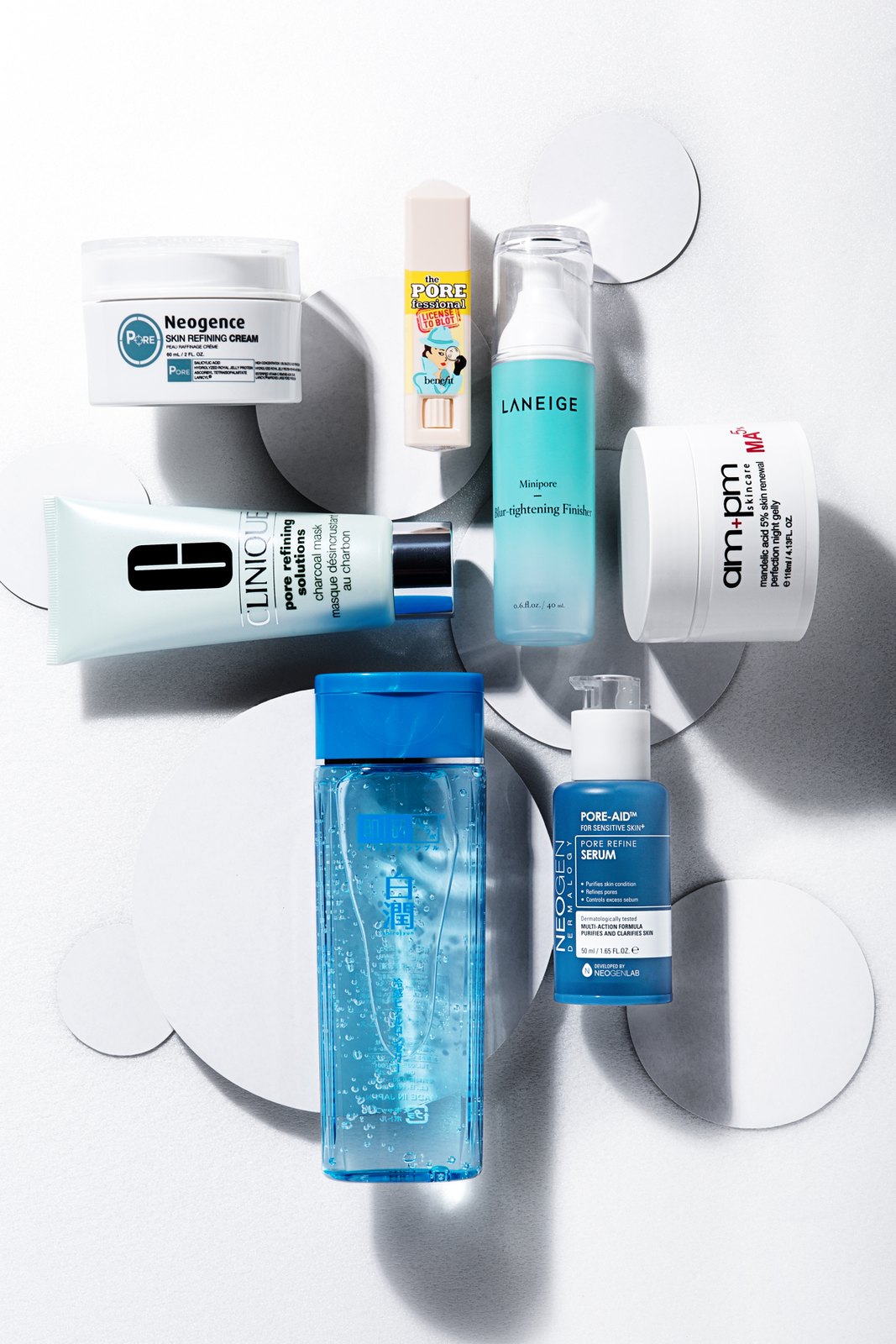This photograph showcases an artistic flat lay arrangement of various skincare and face-cleaning products, meticulously positioned on a pristine white background. Interspersed among the products are paper or card circles of varying sizes, adding an element of visual interest to the layout. 

The light source, originating from the upper left, bathes the top left corner in bright light, creating pronounced shadows that add depth and dimension to the composition. The products, predominantly white and shades of blue, are thoughtfully placed in a clockwise pattern.

- At the midpoint on the left is a Clinique product, recognizable by its sleek design.
- Moving clockwise, there is a Neutrogena product housed in a small white tub.
- Next, there is a boxed item containing a tube, though the brand name is not visible.
- Following this, a Laneige product, identifiable by its turquoise blue tube with a clear lid, catches the eye.
- At the four o'clock position, an ANPM cream is presented in a white tub.
- Around the five o'clock mark, a small bottle filled with blue liquid features a white lid.
- Finally, at the six o'clock position, a clear plastic bottle containing blue liquid rounds out the meticulous arrangement.

This carefully curated display highlights the elegance and simplicity of face-cleaning products through a sophisticated use of color, light, and strategic placement.